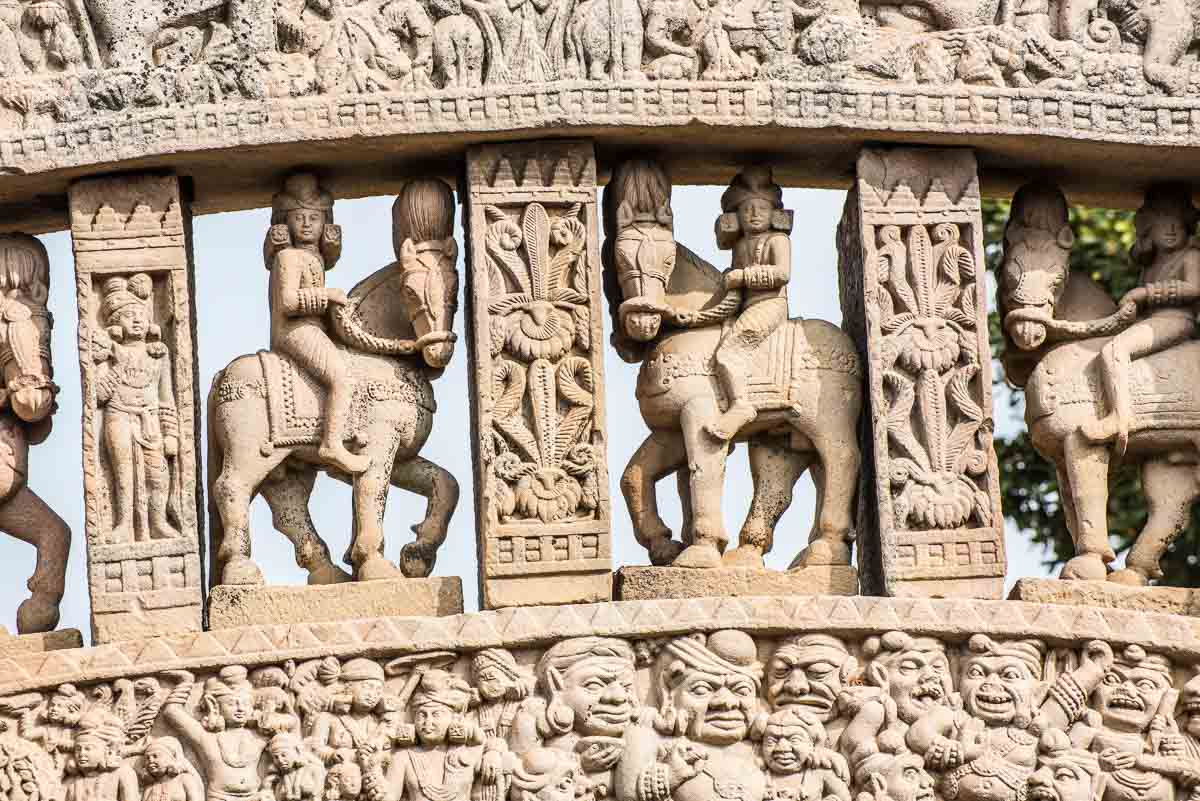The image is a color photograph showcasing an intricately carved stone or cement wall, possibly part of an ancient monument or building. The wall, in an off-white sand color with hints of brown, stands against a backdrop of a light blue sky, with green and yellow tree leaves visible on the far right. The centerpiece of this structure is a series of detailed carvings: at the top, a checkerboard pattern of decorations is distinctly visible. Beneath this, sequences of riders on horseback are flanked by columns, with each segment displaying carefully etched figures. 

In the middle section, a column of swords adds to the symmetry, followed by another segment of horse riders. Along the bottom of the wall, a line of triangular designs stretches horizontally, below which is a remarkable array of 3D faces and figures. These faces vary significantly; some portray deities or characters with serene or peaceful expressions, while others appear monstrous, impish, or are making exaggerated, crazy faces. The overall craftsmanship is highly intricate, reflecting a blend of mythological and possibly cultural motifs, suggesting it could originate from an historical site in Asia, potentially Mongolia or China. The scene contains no readable text and, despite the speculation, it's undetermined whether the photo was taken professionally.